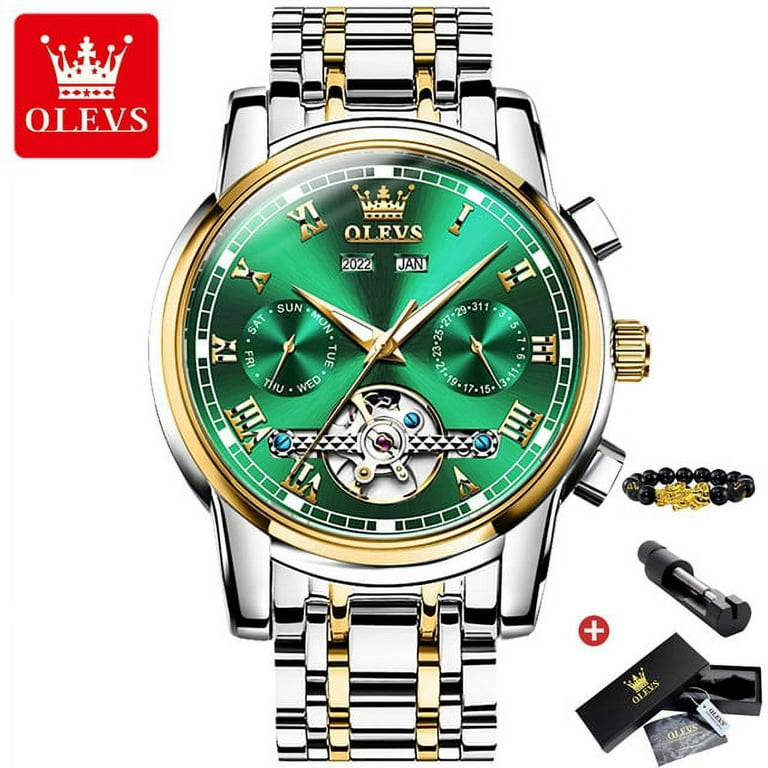This image features an advertisement for a luxurious OLEVS watch set against a clean white background. In the top left corner, the logo is prominently displayed within a red box, featuring a white crown design and the brand name "OLEVS" beneath it. The watch itself, showcased centrally, exudes elegance with its combination of silver and yellow gold. The band is silver with gold stripes running through the center, while the bezel features a gold rim encircling its silver edge. Its striking emerald green face is adorned with luminescent gold Roman numerals, gold hands, and blue accents, including screws at the bottom. Additionally, the watch's face bears gold and blue details that enhance its sophisticated design. To the right of the watch, several accessories are included: a sleek black bead bracelet, a black case marked with a gold crown emblem, and tools presumably for adjusting the watch links. This comprehensive set emphasizes both the luxurious and practical aspects of this timepiece.